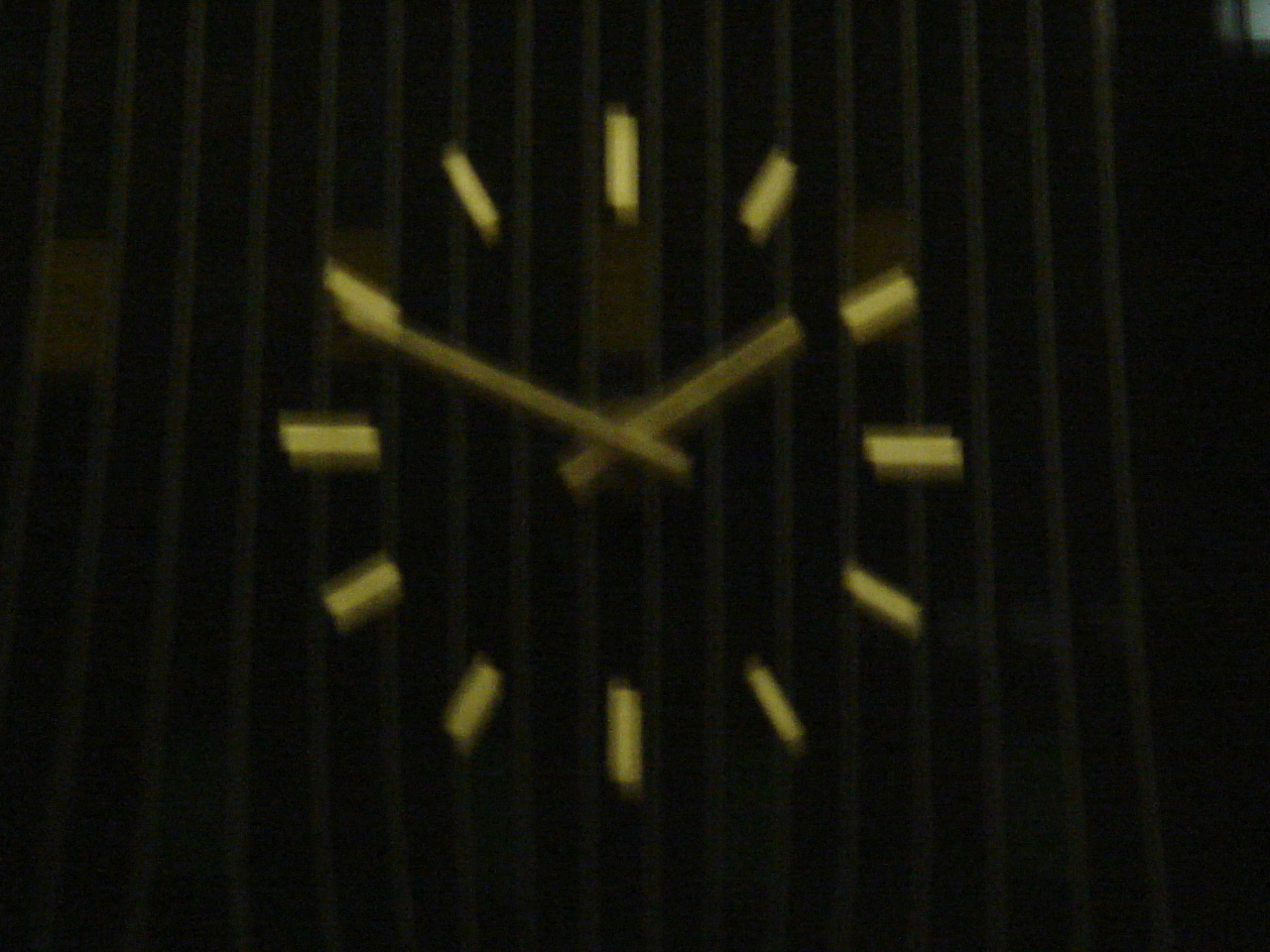This grainy and blurred image shows an interior scene captured through vertical blinds within a dimly lit room. The vertical blinds appear gray due to the low lighting. Beyond the blinds, a black wall is visible, though it isn't uniformly dark, showing subtle variations in shading. The focal point of the image is a golden-highlighted wall clock mounted on the black wall. The clock, devoid of Roman numerals or numeric numbers, features only gold hour indicators and two gold arms – an hour hand and a minute hand. The clock displays 1:50.